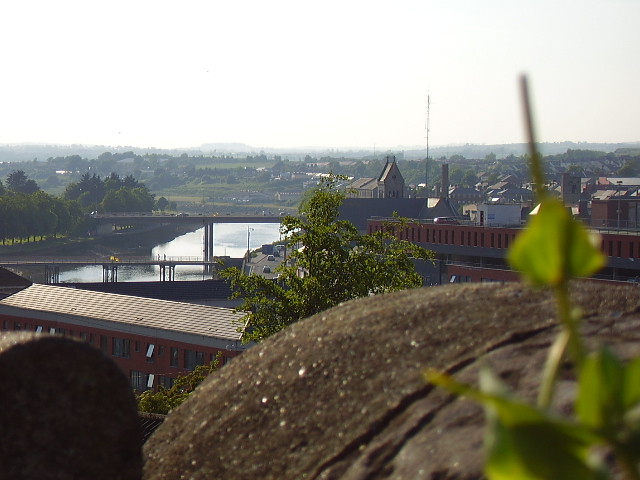This detailed image depicts a landscape view of a city from a distance, likely taken from an elevated position atop a hill. The picture is vertically rectangular, with the top portion being mostly overcast sky, giving a slightly white, cloudy appearance. The cityscape primarily occupies the right side of the image, showcasing a cluster of low-rise buildings, some as tall as two stories, set against a backdrop of distant hills and a mountain range further back.

In the foreground and extending to the left side, we observe expansive fields bordered by lush, dark green tree lines. There are also noticeable man-made infrastructures such as bridges and parking lots, with some cars visible. A river meanders from the left towards the center, where it appears to flow into the urban area, possibly spanned by a bridge. The left side along the riverbank features more natural elements, including greenery and shrubberies. A large, barren hill composed of soil and dirt stands out prominently in this mixed natural and urban scenery. In the far left corner, a yellow object or possible signage is faintly discernible, adding a touch of color to the predominantly green and urban tones.